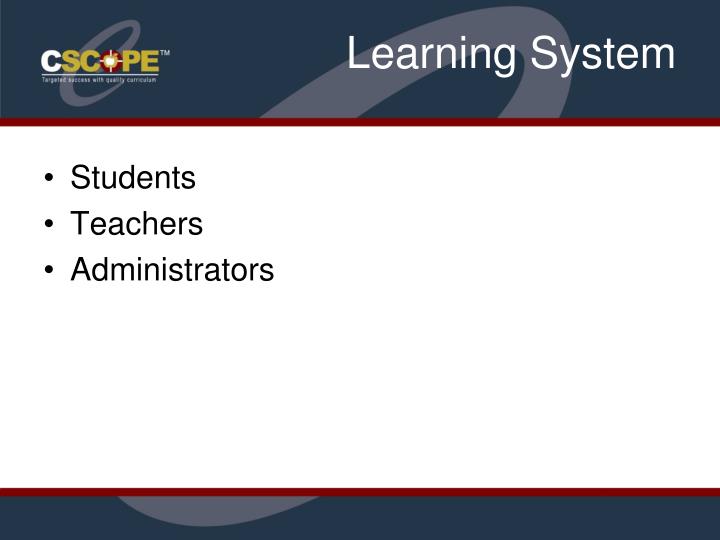This image is a detailed presentation slide designed for an educational purpose, featuring a combination of text and graphic design elements. The background is mostly white with structured horizontal bands at the top and bottom in dark navy blue, creating a clean and formal look. At the very top, there's a gray horizontal band with a distinctive swash of a 'C' visible in a light white tint, part of the C-SCOPE logo. This logo, positioned in the upper left corner, comprises a white 'C', with the letters 'S', 'C', 'P', and 'E' in gold, and a star shape between the 'C' and the 'P'. Opposite the logo, in the upper right corner, is the title "Learning System" in white text.

The central area of the slide contains the main body of text, which includes three bullet points in black, listing "Students," "Teachers," and "Administrators." These points are positioned slightly to the left, ensuring balance and readability. The layout is completed with another strip at the bottom resembling the top design, tying the overall aesthetic together and emphasizing the infographic style of the presentation. The colors used throughout include dark blue, gold, white, gray, red, black, and burgundy, contributing to a visually appealing yet informative slide.